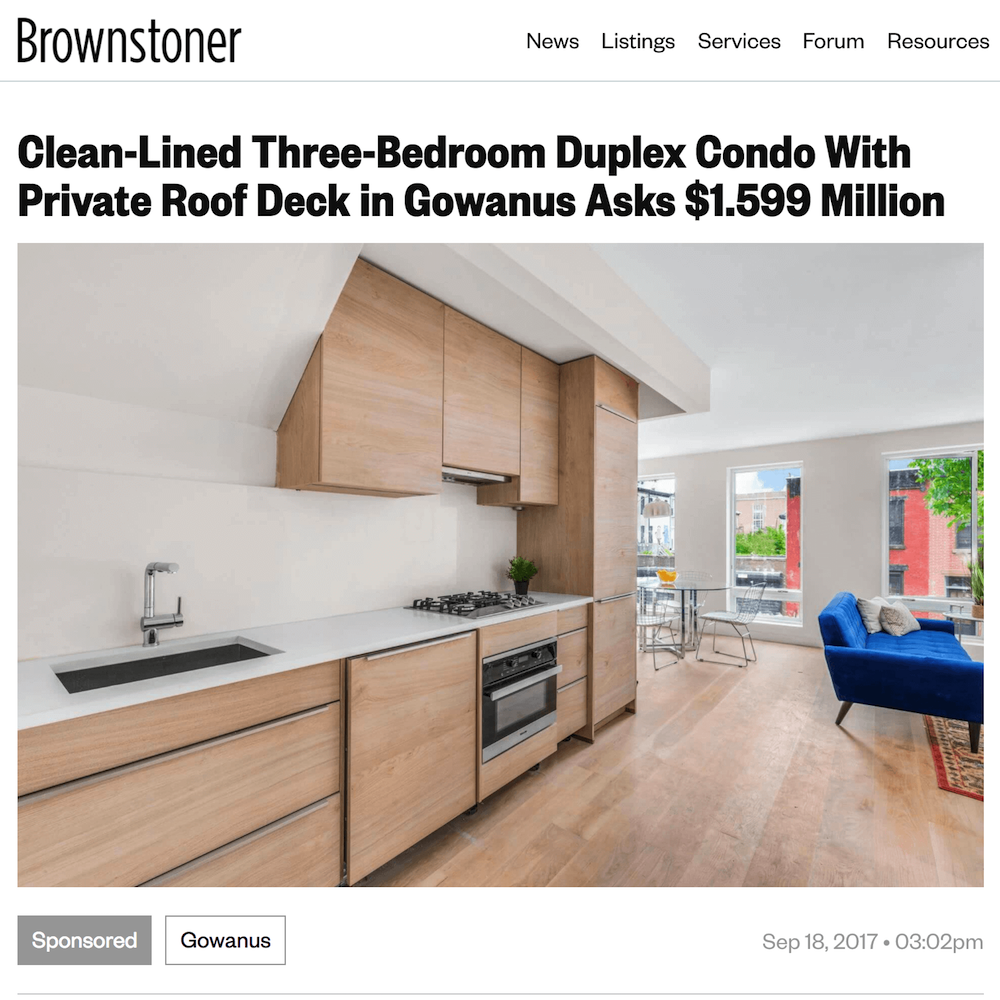The image is a screenshot of a real estate listing from the website Brownstoner. At the top, a white header displays the stylized website name "Brownstoner" in big black text on the left. On the right side of the header, smaller black text lists menu items: "News," "Listings," "Services," "Forum," and "Resources," with spaces between each. Below this, a gray horizontal line divides the header from the listing's title. The title, in bold black text, reads: "Clean-lined three-bedroom duplex condo with private roof deck in Gowanus asks $1.599 million."

At the very bottom of the page, there are two buttons. The first, on the left, is a rectangular gray button with white text that reads "Sponsored." The second, beside it, is a white-bordered gray button with black text that reads "Gowanus." To the extreme right at the bottom, light gray text indicates the date and time of the listing: "SEP 18, 2017, 3:02 PM."

The center of the page features a prominent image of the property. The kitchen, styled with wood and white finishes, is the focal point. Windows and a dining room are visible in the background, suggesting a spacious and well-lit interior.